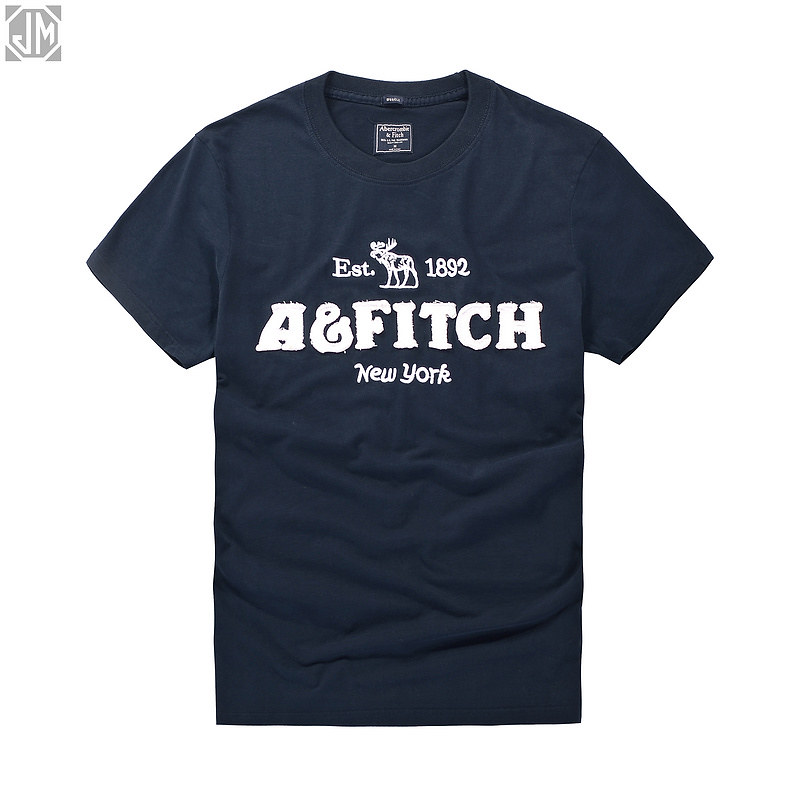The image features a dark blue short-sleeve t-shirt with a crew neck laid flat, highlighting some natural wrinkles in the fabric. Prominently displayed across the front of the shirt is a series of white text and graphics. At the top, it reads "EST." followed by a white illustration of a moose, and the year "1892" beneath it. Below this, in bold white cloth letters, it states "A&Fitch," with "New York" written in smaller white letters underneath. The shirt also includes a blue tag inside the collar with white writing, indicating its brand, Abercrombie & Fitch. The background is white, and there is a gray "JM" logo in the top left corner of the image. The text and logo on the shirt appear to be details stitched from separate cloth pieces rather than simply printed on the fabric.